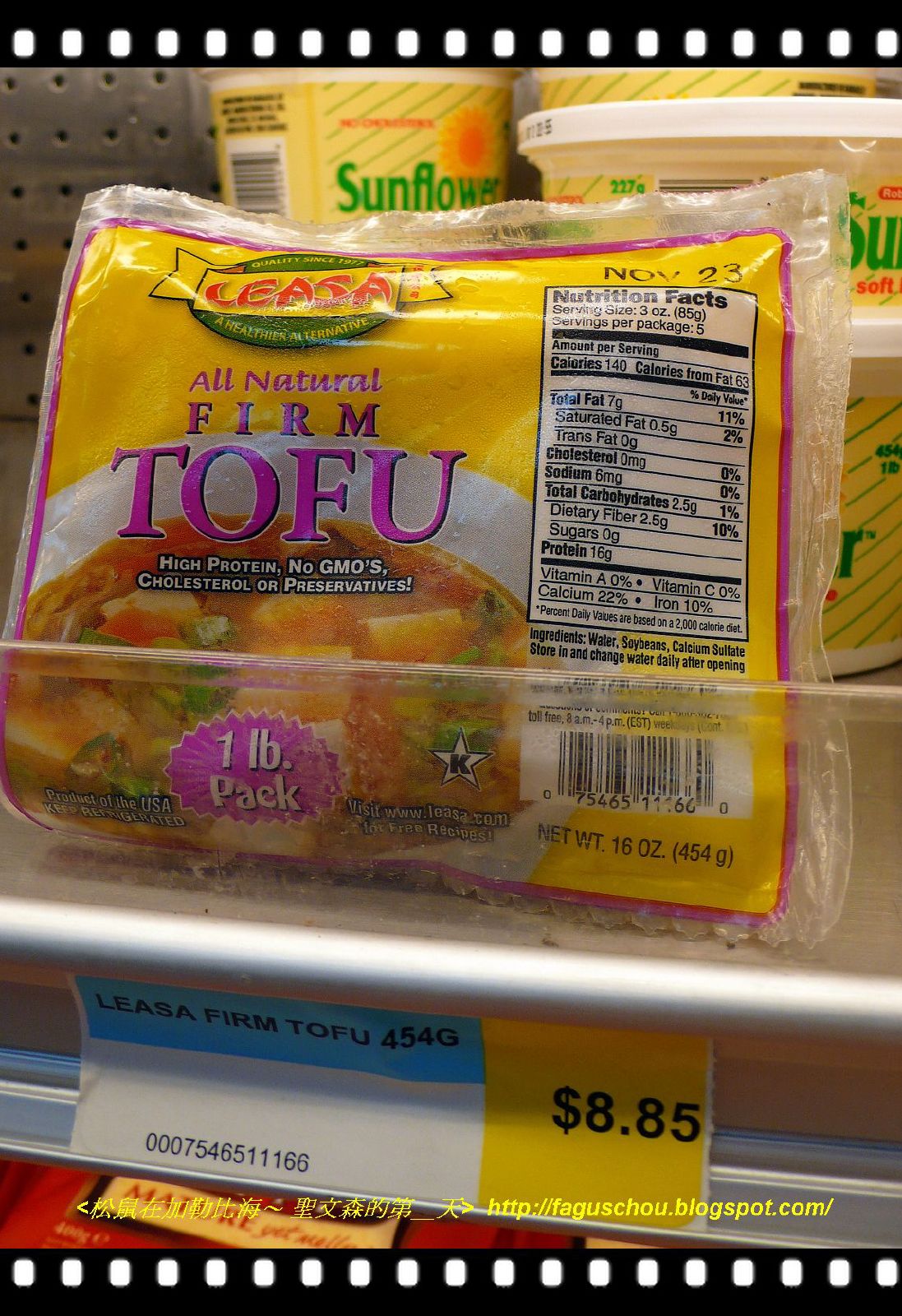This detailed photograph captures a single yellow package of Lisa (L-E-A-S-A) all natural firm tofu on a refrigerated shelf in a grocery store. The tofu, clearly marked with "high protein, no GMOs, cholesterol or preservatives," is housed in a one-pound (16 ounces/454 grams) pack with visible nutritional facts on the front of the package. The tofu's packaging appears to have condensation on it, indicating it is well-chilled. Below the tofu is a price tag on a standard silver bar, reading $8.85. Positioned in a cooler rack, the tofu seems to be the last package on the shelf, with products labeled "Sunflower" visible behind it, likely margarine tubs. A link to a blog, faggoshow.blogspot.com, is noted towards the bottom of the package, along with some Asian characters. The bright pink text and image of soup with floating tofu on the packaging add a vivid contrast to this neatly arranged store display.